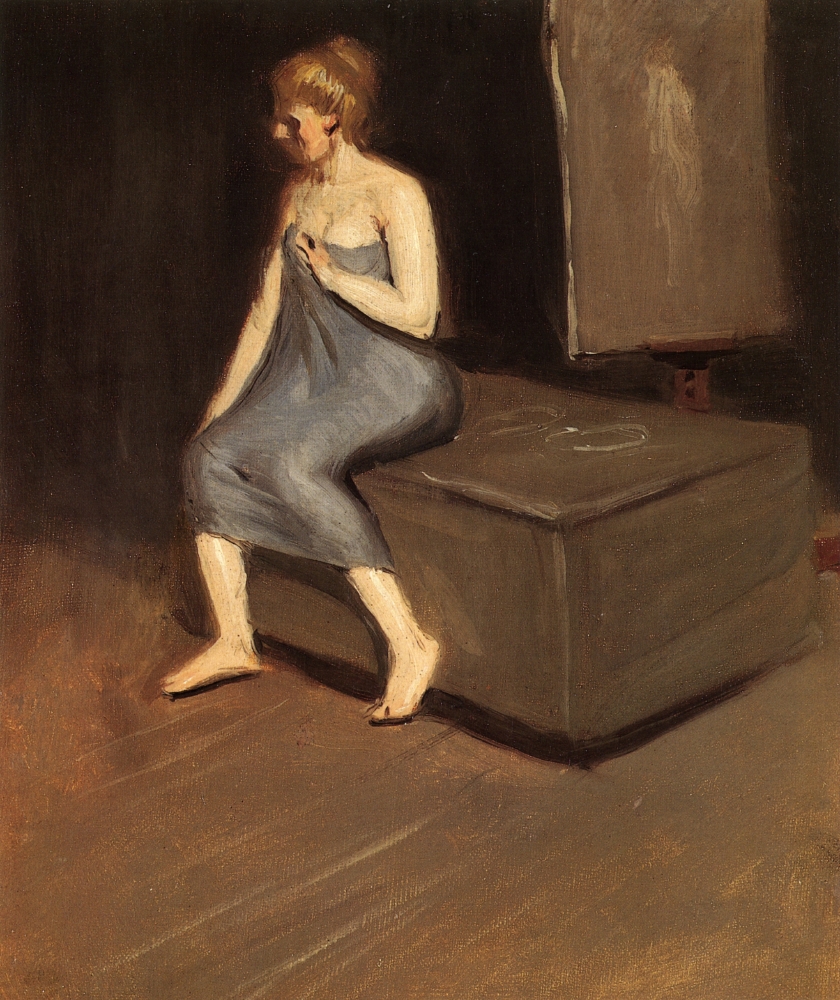The image is an almost square artwork, slightly taller than it is wide, depicting a light-skinned woman sitting barefoot on a three-dimensional, dark grayish-brown rectangular box. The background is predominantly black with a lighter grayish-brown rectangular shape on the upper right, possibly suggesting a window. The floor appears to be made of wood with a brown color. The woman, with chestnut brown hair styled in a bun, is draped in a dark gray cloth or towel that wraps around her chest and extends to just below her knees. She faces towards the left side of the image, with her facial features indistinct.